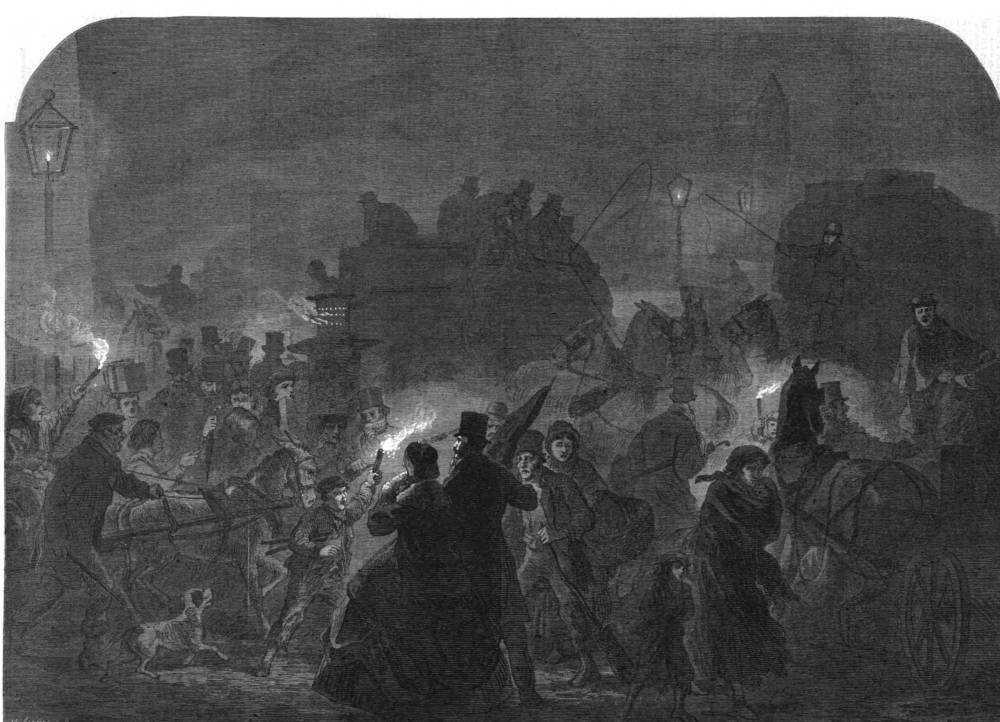This black-and-white image, which appears almost like a sketch, captures a bustling, historical street scene reminiscent of early 1900s England. The streets are alive with a large crowd, predominantly men in old-fashioned pants and jackets, and a few women donning petticoat dresses. The scene is dotted with barking dogs and the occasional horse-drawn carriage, hinting at a time before automobiles became widespread. Street lamps, fueled by gas, illuminate the atmosphere while a few individuals carry torches, adding to the sense of an eventful gathering. The indistinct yet tall and triangular building facades in the background enhance the European vibe of the setting. Notably, one figure, dressed in a striking top hat, resembles Abraham Lincoln, contributing to the depiction's evocative historical ambiance.